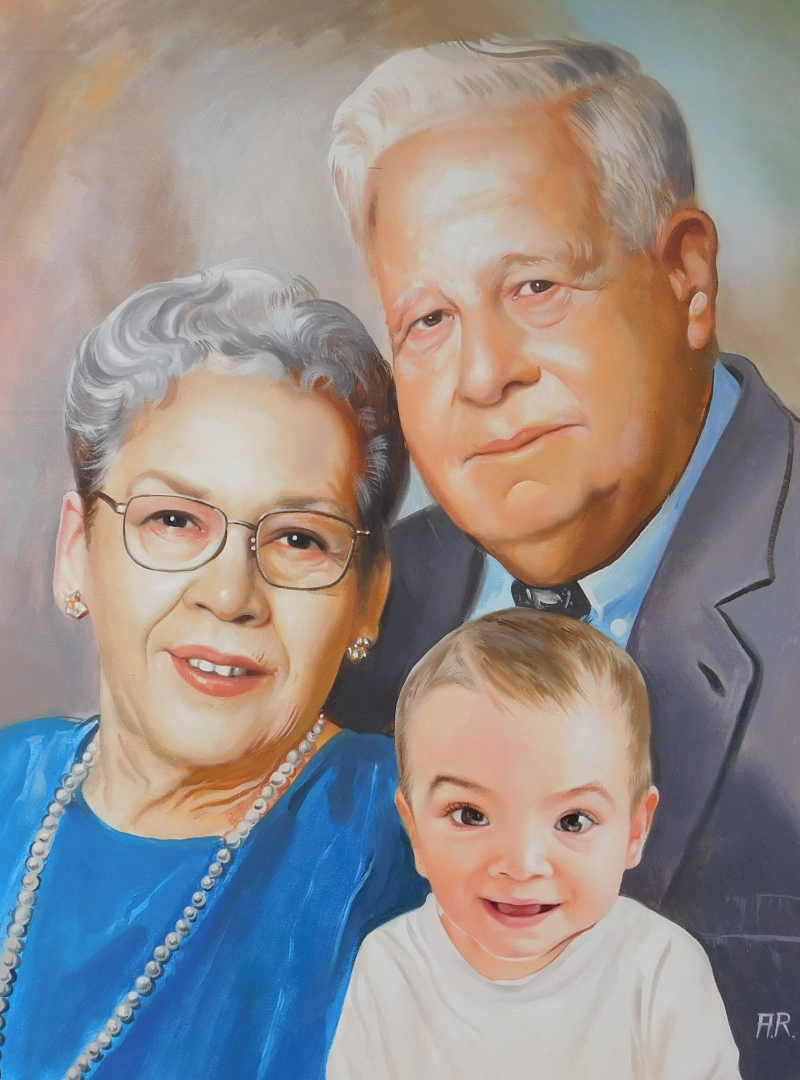This portrait, rendered in an oil painting style with a semi-photorealistic touch, features three individuals against a background of swirling browns, grays, and beiges. On the left is an elderly woman with short gray hair, rounded rectangular glasses, and a pearl necklace. She has red lipstick, diamond stud earrings, and wears a blue dress, smiling softly with her mouth slightly open. To her right, positioned slightly behind, is an older man with short white-gray hair combed back. He has a tall forehead and a long, thick face, dressed in a gray blazer, blue shirt, and dark tie. He too gazes directly ahead with a subtle smile. In the center foreground is a light-skinned baby in a white onesie, with short brown hair and dark eyes wide open, smiling at the viewer. The initials “A.R.” are painted in the bottom right corner. The painting conveys a sense of familial warmth and connection, encapsulating the essence of a multigenerational family portrait.